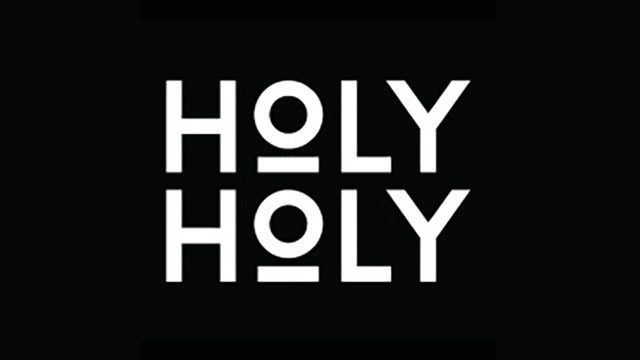The image is a horizontally oriented black rectangle featuring two identical lines of text in the center, both reading "HOLY" in large, white sans-serif font. The letters are evenly spaced, and each "O" has a thin, horizontal underline beneath it, adding an unusual emphasis. The top row of "HOLY" is directly above the second, creating a simple but striking visual repetition. The minimalist design focuses entirely on the repeated word "HOLY," underscored by the unique underlining of the "O," likely intended to draw attention or convey a specific, yet mysterious, message.